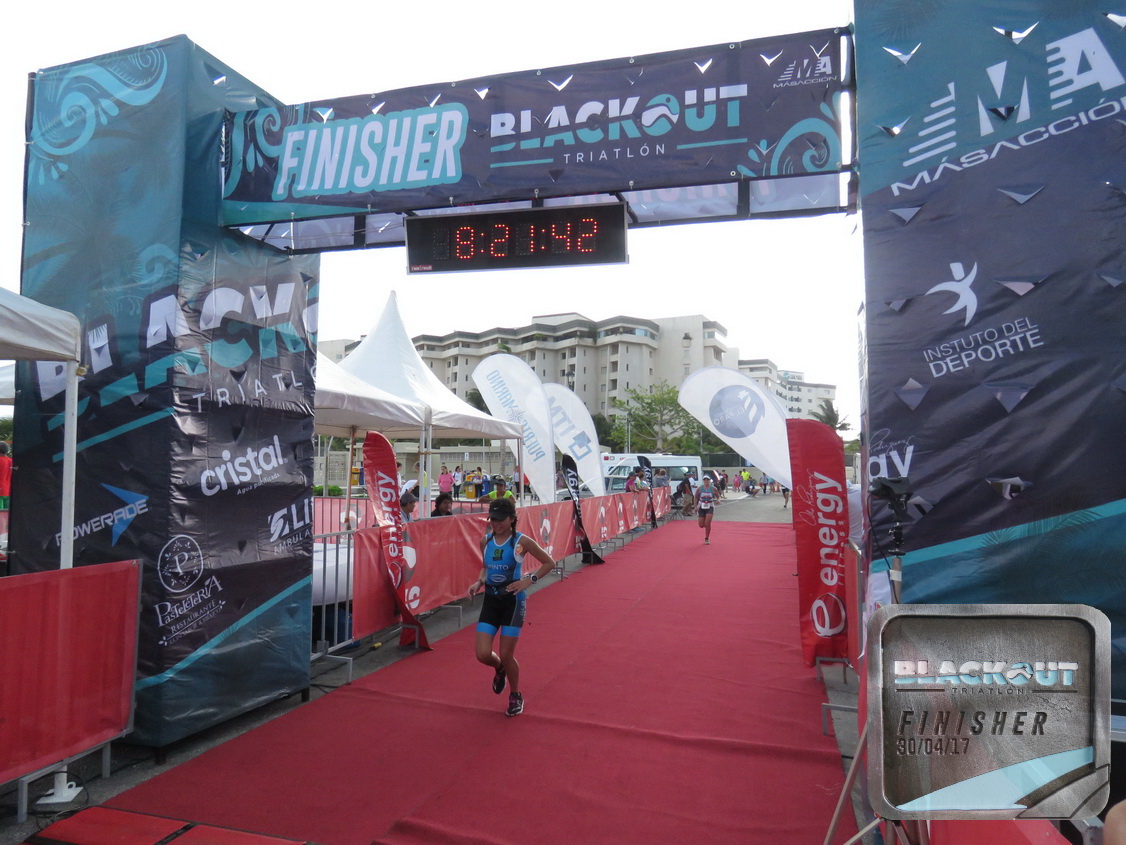In this detailed photograph, we see the vibrant finish line of the Blackout Triatlón, likely set in a foreign country, as indicated by the spelling "Triatlón" with an accented "O". The foreground captures a momentous scene where a female runner, dressed in a blue running uniform and a black cap, is crossing under an archway festooned with sponsor logos such as Powerade, Crystal, Pastelateria, and Instituto del Deporte. The digital clock above her displays a time of 8 hours, 21 minutes, and 42 seconds. The word "Finisher" is prominently displayed at the top of the arch, affirming this is indeed the finish line. The runner ahead is followed by another female competitor; both are making their way over a striking red carpet that marks this final stretch. The backdrop reveals additional runners approaching the finish line, progressing on the regular pavement. The entire scene is bathed in daylight, despite the heavy overcast, hinting at a resort-like villa or hotel setting in the background. On the left side of the arch in the image, concession stands add to the bustling atmosphere, rounding out this vivid portrayal of an exhilarating race conclusion.